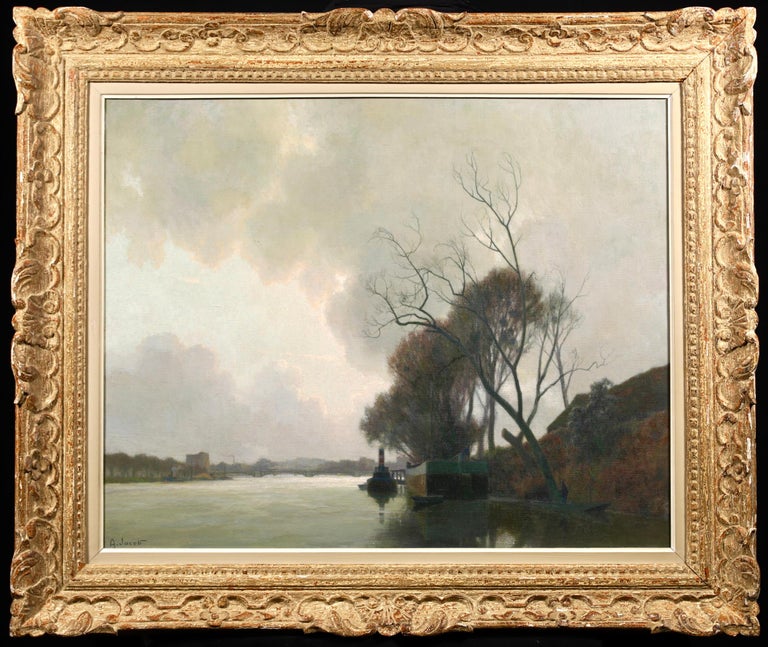This image presents a photograph of a framed, traditional style landscape painting, encased in a highly intricate and ornate gold-gilded frame with multiple layers of detailing, including a thick outer frame and dual inner mats—a thin beige and a tight white one. The painting itself depicts a serene, cold day at a lake or possibly a slow-moving river. The foreground features a hilly range or cliff descending towards the water, adorned with large, leafless trees, hinting at an early winter or late fall setting. The sky is gray and cloudy, subtly lined with pinkish light where the sun attempts to break through. In the water, there is at least one boat, seemingly just having taken off from a landing, steering toward the horizon. The background includes some indistinct buildings and what might be bridges, cloaked in a hazy pastel atmosphere, contributing to the tranquil and somewhat melancholic mood of the scene.